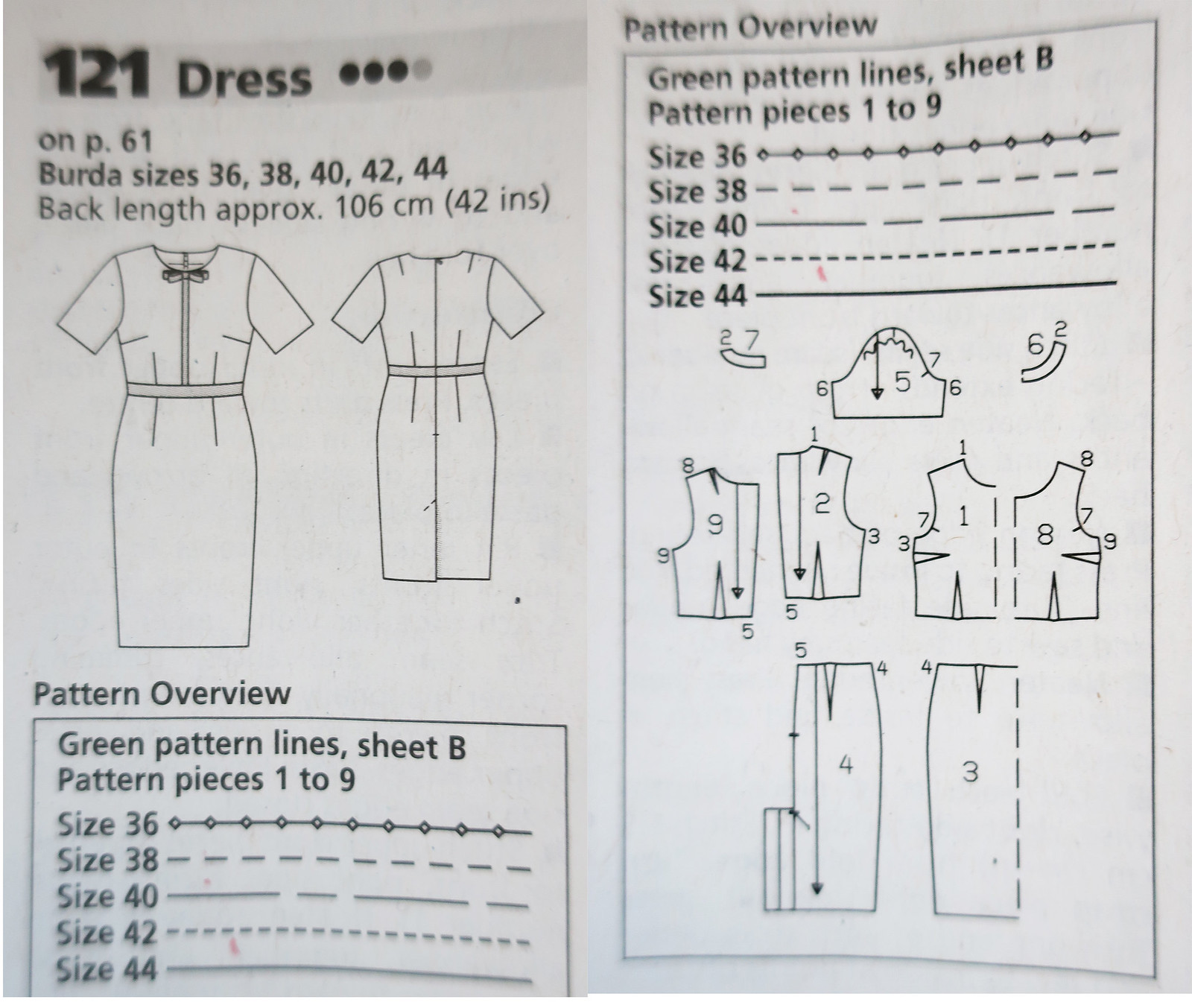This image is a detailed scan of a sewing pattern for the "121 Dress" found on page 61. The left side prominently displays "121 Dress" along with Burda sizes 36, 38, 40, 42, and 44, specifying a back length of approximately 106 centimeters (42 inches). Below this, a front and back view drawing of the dress is shown. A "Pattern Overview" section follows, indicating that the pieces are on the green pattern line, sheet B, covering pattern pieces 1 to 9 for the listed sizes. The right side repeats these details with an emphasis on the pattern's breakdown, showing different segments of the dress, each numbered. The background is white, with some areas appearing lighter.